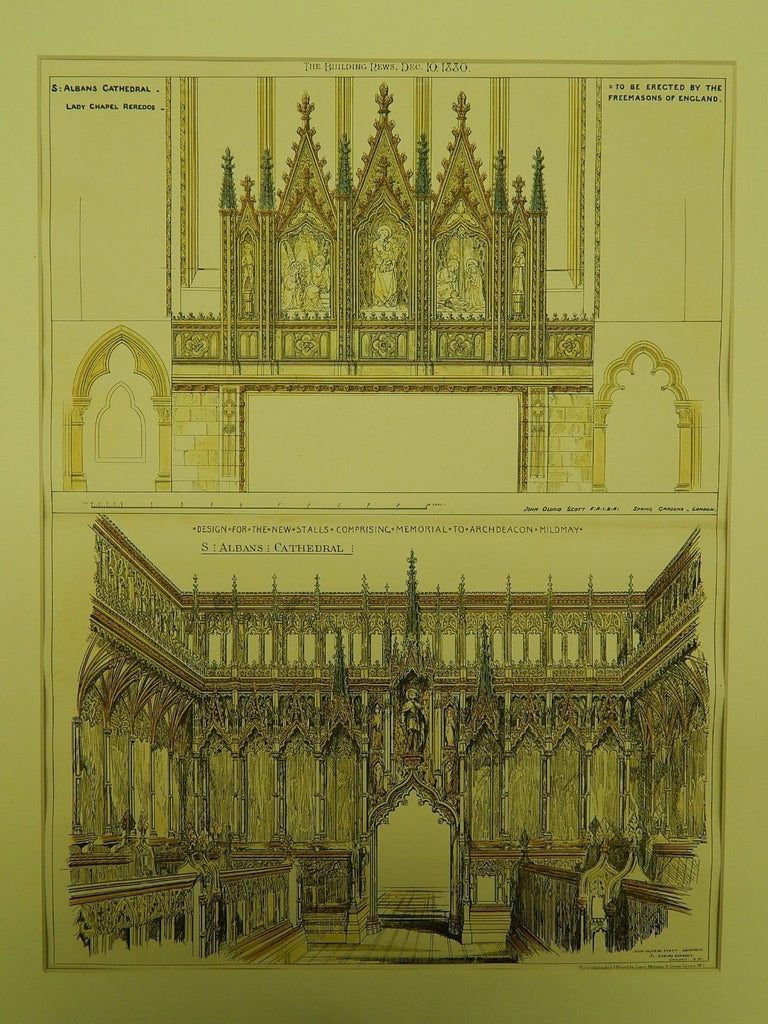This image appears to be a detailed architectural drawing or diagram of St. Albans Cathedral, specifically the Lady Chapel. The illustration, which has a yellow tint, includes ornate sketches resembling blueprints. In the top left corner, the text reads "St. Albans Cathedral, Lady Chapel, Reredos to be erected by the Freemasons of England." The upper right section contains a similar notation, "Designed for the new stalls comprising memorial to Archdeacon Malleolme." Additionally, there's a date inscribed: December 10th, 1880. The drawing meticulously depicts the interior, highlighting pews, a beautiful arched doorway resembling the top of icing on a cupcake, stained glass windows, and what seems to be the altar. The illustration fills a large rectangular space and gives the feeling of a page from an architectural or historical book.